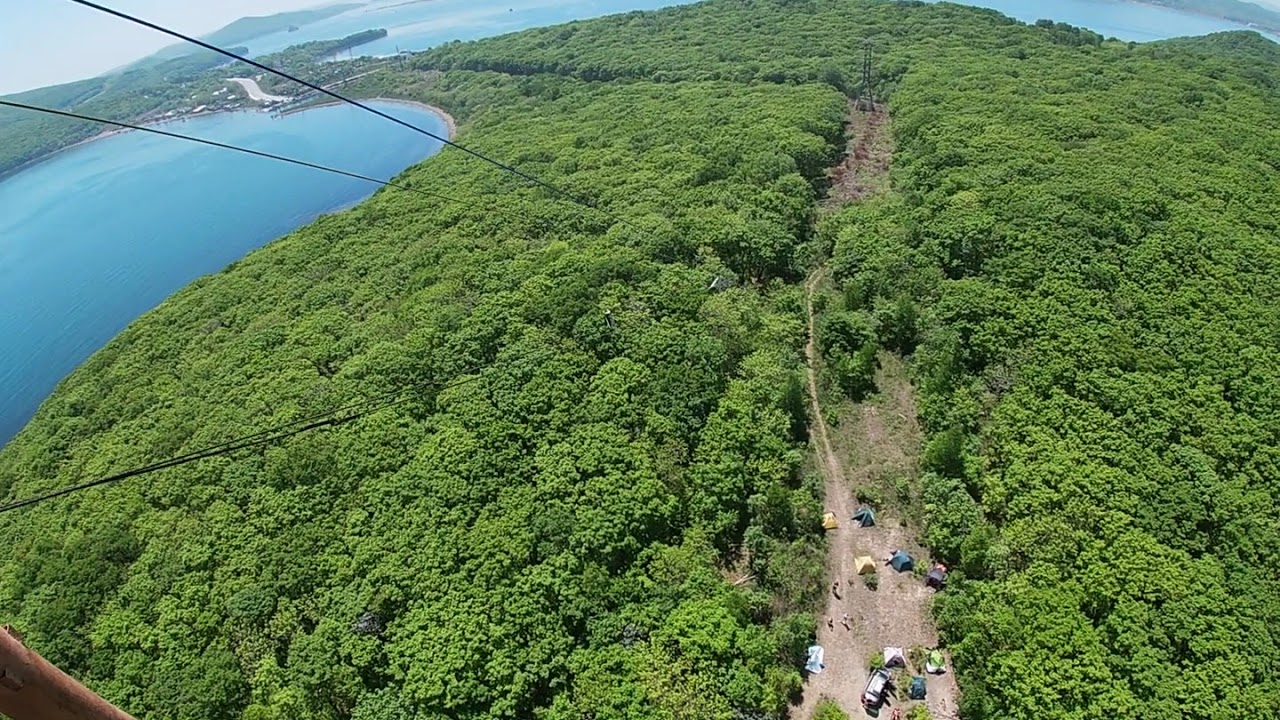The photograph, taken from a high vantage point such as a tower, drone, or cable car, captures a broad aerial view of a verdant landscape. In the lower left corner, a brown object, likely part of a pole, is visible, from which black lines or wires extend downwards. From this elevated perspective, a vast forest of predominantly deciduous trees stretches out, tapering into a small clearing in the middle. This clearing is dotted with tents, vehicles, and a few discernible people. A dirt road weaves through the dense foliage, leading towards bodies of water visible on both the left and distant horizons. The left side of the image particularly features a body of water, possibly a bay or lake, with more water faintly visible in the upper right-hand corner as well. The scene is bathed in bright sunlight, casting a cheerful light over the lush greenery, and there are mountains faintly visible in the distance, adding depth to the expansive natural setting.